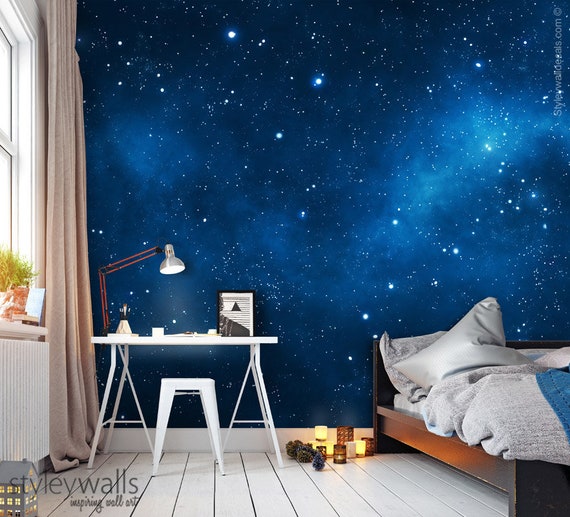This image is an advertisement for Stylieville Walls, featuring their "Inspiring Wall Art." The central focus of the photo is a bedroom with a captivating blue galaxy mural on the wall, depicting swirling hues of blue and numerous stars with no planets. The scene portrays a modern yet cozy atmosphere. In the bottom left corner, dark gray text reads "Stylieville Walls, Inspiring Wall Art," and additional branded text runs upwards in the upper right corner. The room is minimally furnished, drawing attention to the impressive wall art.

A low, dark wooden bed with disheveled tan blankets is positioned near the center of the image. Beside the bed on the floor, there are candles emitting a soft yellow glow and inexplicably, some pine cones scattered around. Adjacent to the bed is a small, contemporary white desk with a metallic lamp and a stool. The desk holds a few objects, including a framed photo. To the far left, a tan full-length curtain covers a window, which has several plants on the sill, adding a touch of greenery to the space. A radiator or possibly a miniature house-like object is also discernible near the window. The flooring is whitewashed wide wooden planks with a rustic finish, enhancing the room's aesthetic.